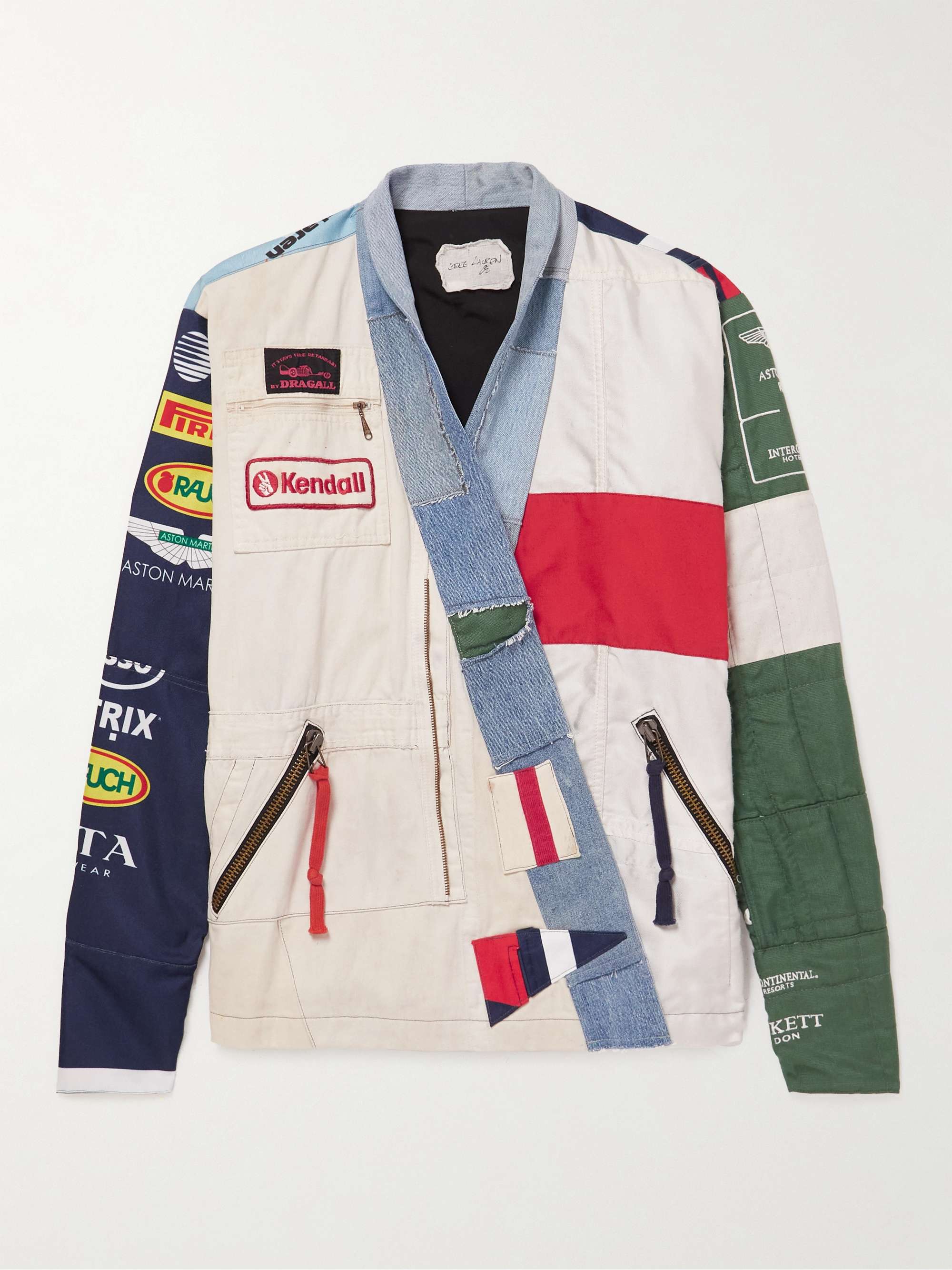The photograph captures a uniquely styled, multi-colored jacket set against a plain white background. The garment is predominately white with a distinct kimono wrap-style closure crafted from denim, eliminating the need for zippers or buttons along the main fastening. Across the chest on the left side, a prominent red patch replaces the traditional pocket location, while two diagonal zipper pockets, one with a blue zipper pull and the other with a red pull, feature on the front. An intricately detailed label with the Kendall logo adorns the front, adding to its varied charm.

The jacket’s right sleeve is a dark navy blue, embellished with multiple logos including an Aston Martin patch, a white AT&T logo, a yellow Pirelli logo, and a Raj logo with a red stripe. The left sleeve contrasts sharply in British Racing Green and incorporates a white patch across the bicep, with another Aston Martin logo barely visible on the shoulder. The jacket's blending of colors, patterns, and racing-related patches suggests it might be inspired by the attire of a race car driver, making it a striking, eclectic piece.